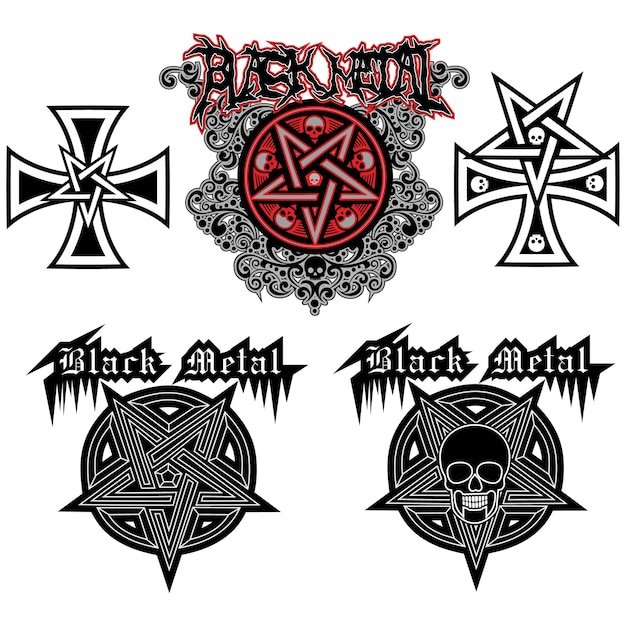The image showcases five emblematic patches arranged with three on the top row and two on the bottom row. At the top, bold black text with a red outline reads "Black Metal." Each emblem is intricately designed, reflecting gothic and metal themes. 

- The top left emblem features a white-bordered black cross with four legs, interspersed with a central black star.
- The top middle emblem comprises a red circle with a red pentagram, accented by swirling patterns and small skulls around the periphery.
- The top right emblem displays a three-legged white-bordered black cross with a star perched at the top tip, and small white skulls embellishing each point.

On the bottom row:

- Both emblems share the phrase "Black Metal" in a spiky font. The left emblem consists of a black circle with a black star superimposed, surrounded by a white border.
- The right emblem is similar but includes an additional black skull with white teeth in the center.

Overall, the emblems blend gothic crosses, stars, and skull motifs, unified under the stark, metallic theme of "Black Metal."